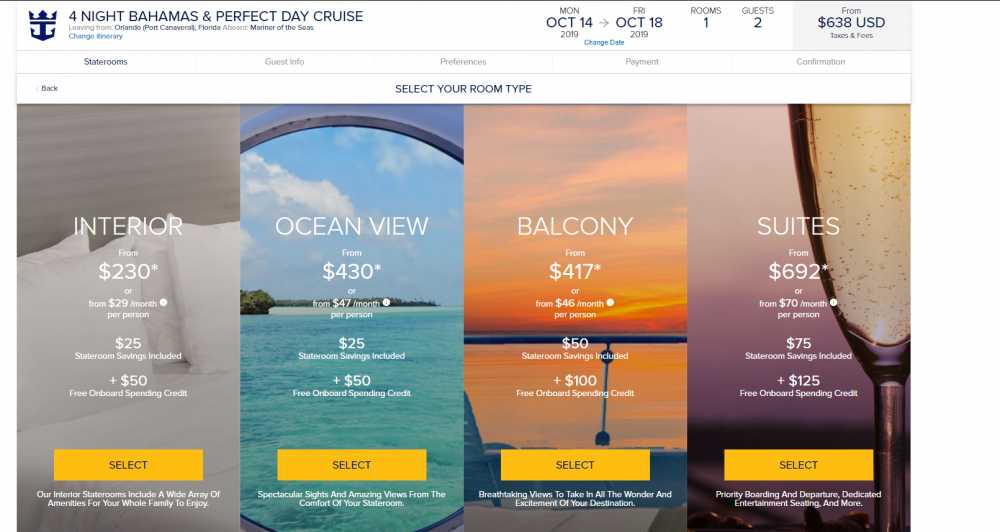This image is an advertisement from a holiday getaway website for a "Perfect Day" Bahamas cruise. The offer is for a four-night cruise scheduled from Monday, October 14th to Friday, October 18th. Currently, one room remains available, and the booking is for two guests at a starting price of $638 USD. The ad presents four room options: Interior ($230), Ocean View ($430), Balcony ($417), and Suites ($692). Each room type is shown with accompanying images to illustrate the accommodation. The room choices are listed in order of increasing price.